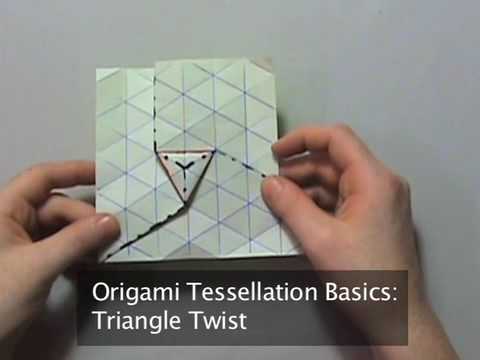This image appears to be a screenshot from a video tutorial titled "Origami Tessellation Basics: Triangle Twist." The background is a grey color, possibly representing a table surface. The image captures a close-up, almost point-of-view shot, of a Caucasian person’s hands holding a piece of paper. The paper is covered with a complex pattern of diagonal lines crisscrossing to form several diamond shapes and sets of triangles. These lines are likely drawn to guide the folding process of the origami design. At the center of the paper, there is a distinctive triangular shape with lines radiating outward at roughly 60-degree angles, indicating the foundational structure of the triangle twist tessellation.